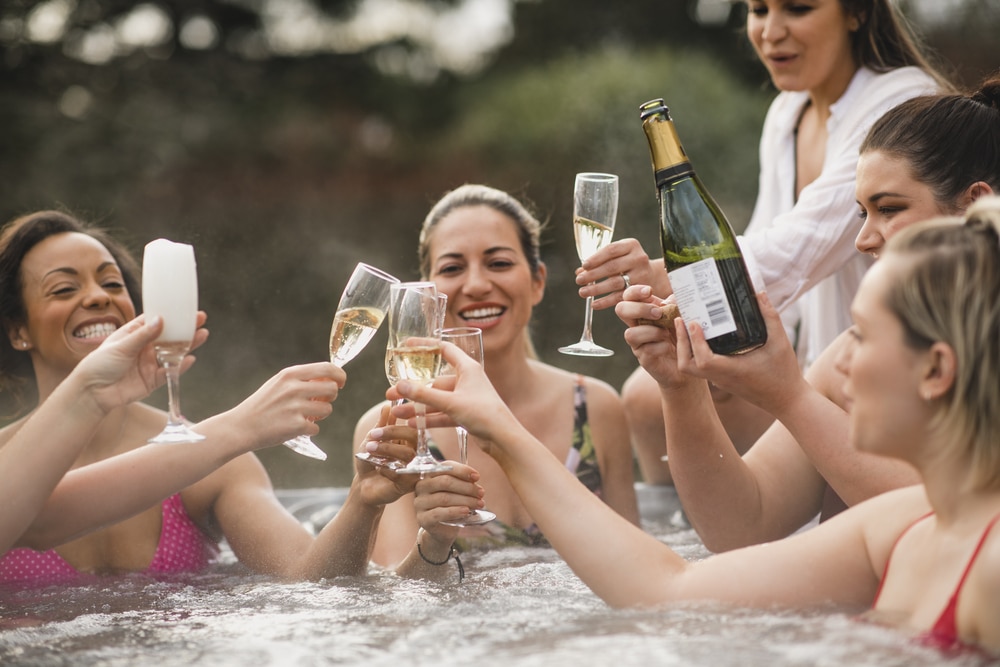In this celebratory photo, five women are seen enjoying a joyous occasion in a hot tub. Four women are immersed in the bubbling jacuzzi, while the fifth woman, clad in a white beach throw or blouse over her swimsuit, sits on the edge. Each woman holds a glass of champagne, actively toasting one another with radiant smiles. Among them, one woman proudly lifts a half-full, green champagne bottle adorned with a gold foil label on the neck. The group sports a variety of swimwear, including two women in pink bikini tops and another in a green camouflage print bikini top. The background hints at an outdoor setting with visible shrubbery and woods, adding to the ambiance of the warm-weather celebration. The steam rising from the hot tub and the additional arms joining the toast suggest more participants off-camera, contributing to the lively atmosphere, potentially for a bridal or baby shower, as suggested by the women's radiant expressions and the festive mood. The women, a delightful mix of different races, are evidently having a terrific time together.